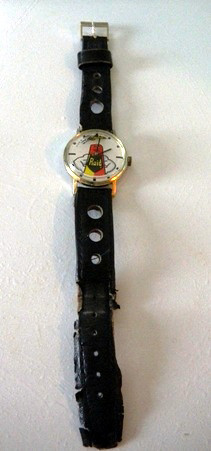In this grainy, low-resolution image, we see a white table or counter bearing a wristwatch laid out horizontally in the center. The watch features a black leather band adorned with small decorative cut-out circles, distinct from the adjustment holes. This black band extends gracefully on either side of the timepiece's white face, which is notable for its minimalist design—a series of black dots marking the hours rather than numerals.

The watch face itself carries an artistic embellishment: a can of Raid Rotary and Spray presented in a pop art style. This illustration, rich with detail, features bold hues of red, yellow, and black, with the word RAID prominently displayed in vibrant yellow letters. The can is bordered in black and a playful cloud outline behind it suggests the iconic spray pattern of the product. The watch shows signs of wear along its edges, adding to its character and hinting at a history of use.